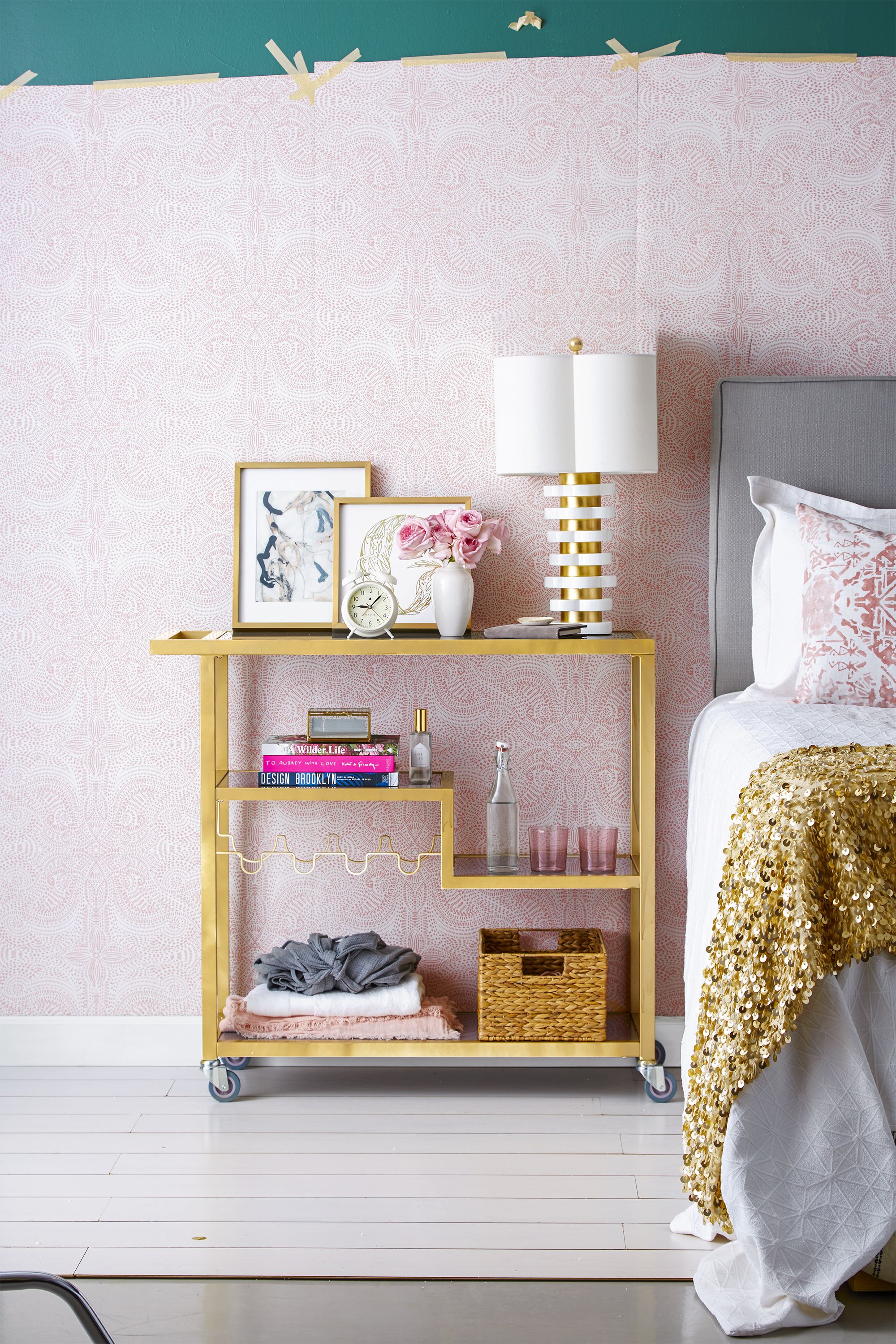The photograph depicts a charming bedroom with pastel hues and intricate detailing. Dominating the left side, the peach-colored wall features a white molding border at the base, blending seamlessly with a plush white carpet. The topmost section of the wall is adorned with a seafoam green border, accented with V-shaped designs matching the peach color. 

The right side of the image includes a glimpse of the bed, characterized by a gray headboard and adorned with white sheets. Pink pillows rest against the headboard, accompanied by a gold or brass covering at the foot of the bed. Adjacent to the bed is a gray, leather-like chair draped with a white cloth edged in gold, hosting a pillow with pink accents. 

To the left of the chair stands a gold or brass cart, which serves as a multifunctional side table. The cart features three shelves: the topmost shelf bears a modernistic two-tone lamp with white accents, a white vase brimming with pink roses, a white alarm clock indicating it is five minutes past nine, and two framed pictures. The middle shelf holds a neat stack of books, a gold-topped bottle of perfume, several small pink glasses, and a bottle of water. Finally, the bottom shelf accommodates a woven wicker basket with two handles, containing folded fabric or clothing.

Every element in the room complements the pastel color scheme, resulting in a cohesive and aesthetically pleasing space.